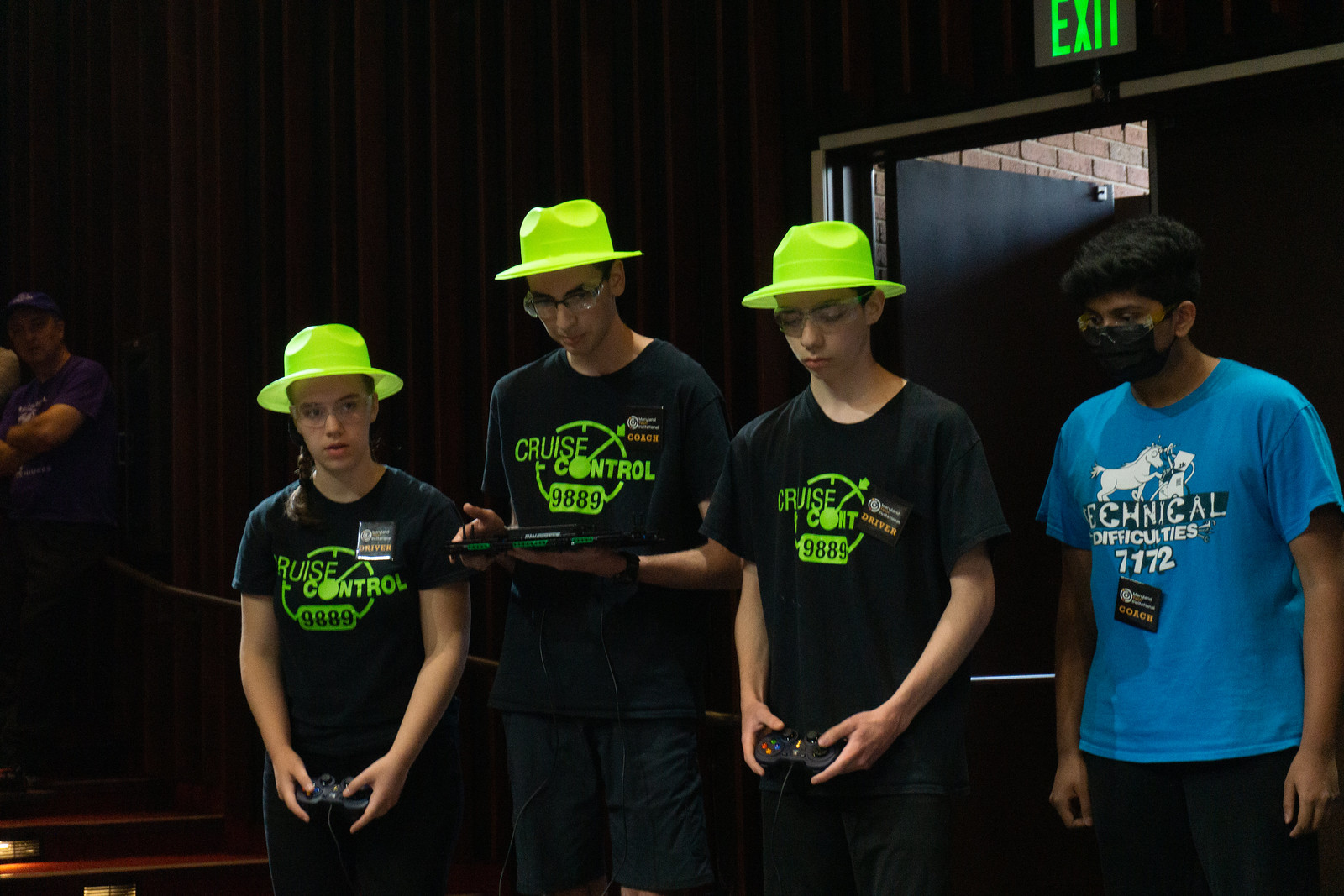In this rectangular photograph, clearly taken during a video game competition, four individuals are standing together inside a hole with a dark ambiance around them. The primary focus is on three team members on the left, who are dressed in matching outfits. They each wear a vivid lime-green top hat, black t-shirts emblazoned with the green text "Cruise Control 9889" that features a circle resembling a speedometer, and badges indicating their roles (likely driver or player). The young woman on the far left, a tall man with glasses in the center, and another smaller man on the right are all holding what seem to be video game controllers. 

To the far right stands a fourth individual, distinct from the team, dressed in a bright blue t-shirt labeled "Technical Difficulties 7172", paired with a black mask and a coach badge, but without a game controller.

The background is a dark, black-walled setting. Behind the group, there is a clearly visible exit door with an illuminated green exit sign above it. Lines on the monochrome wall and the presence of curtains add to the backdrop’s texture. On the left side of the photograph, steps leading upward resemble theater stairs, where a spectator appears to be standing, hinting at an audience beyond.